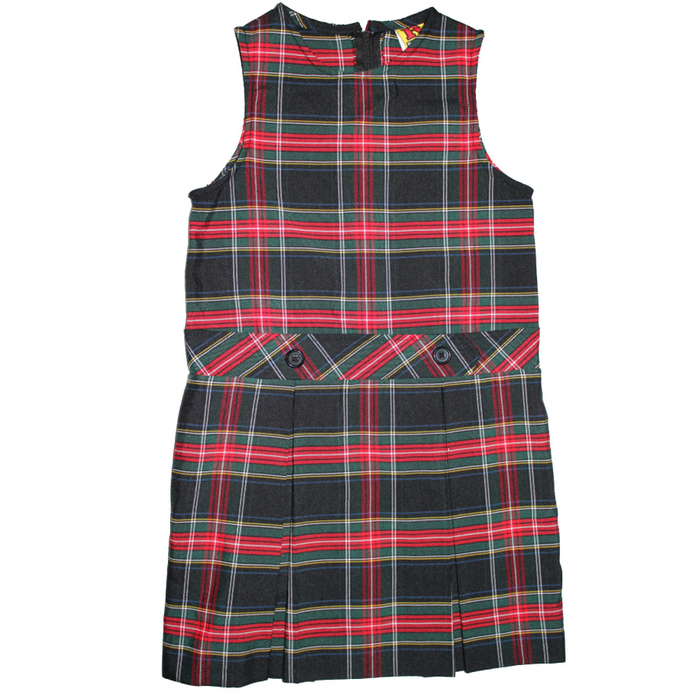This image showcases a meticulously designed patchwork dress, evocative of a school uniform or perhaps a traditional kilt. The dress features a striking combination of black, red, and white colors, with patterns comprising both vertical and horizontal stripes intermingled with red and green patches. The bodice of the dress is sleeveless, enhancing its sleek, modern appearance, and includes a zipper at the top accented by a small yellow tag.

The midsection of the dress, resembling a belt, is crafted from the same patchwork fabric turned diagonally, adding a dynamic element to the design. This section is adorned with two discreet black buttons at the center. The lower part of the dress transitions into a pleated skirt, which enhances its structured and well-tailored look, with the pleats adding a rhythmic, vertical dimension to the silhouette. 

Set against a plain white background, the dress itself stands out, allowing viewers to appreciate the detailed craftsmanship and vibrant color scheme of this unique and potentially symbolic garment.